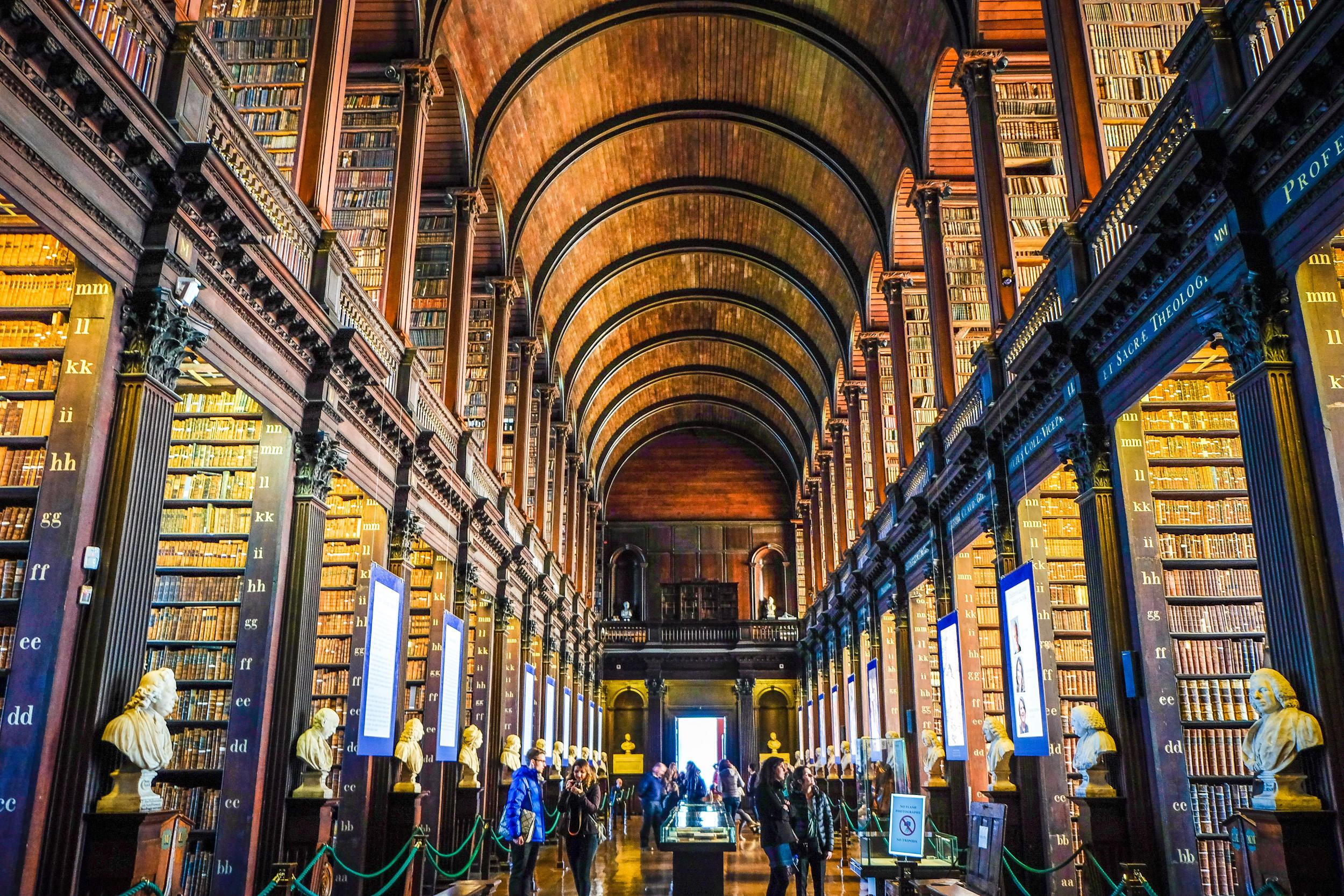The photo depicts the ornate interior of an old, grand library, potentially Trinity College Library. The room showcases a high, arched wooden ceiling that creates a sense of spaciousness. The library features two stories with open balconies on either side, supported by columns and pillars that lead the eye down the central corridor. Floor-to-ceiling bookshelves line both sides of the room, filled with books that have golden and light brown covers. Busts of historical figures, likely authors, are stationed at the entrance of each row of bookshelves. Some areas are roped off with green ropes to restrict access. Visitors appear small in the vastness of the room, contributing to the library's sense of grandeur. Signs on the wooden columns and next to the bookshelves include white markers, possibly indicating sections of the collection. At the far end of the room, the space narrows, drawing focus to either a sign or an open door at the bottom rear, adding to the room's depth and complexity. The intricate detailing and layout reflect the library's rich history and significance.